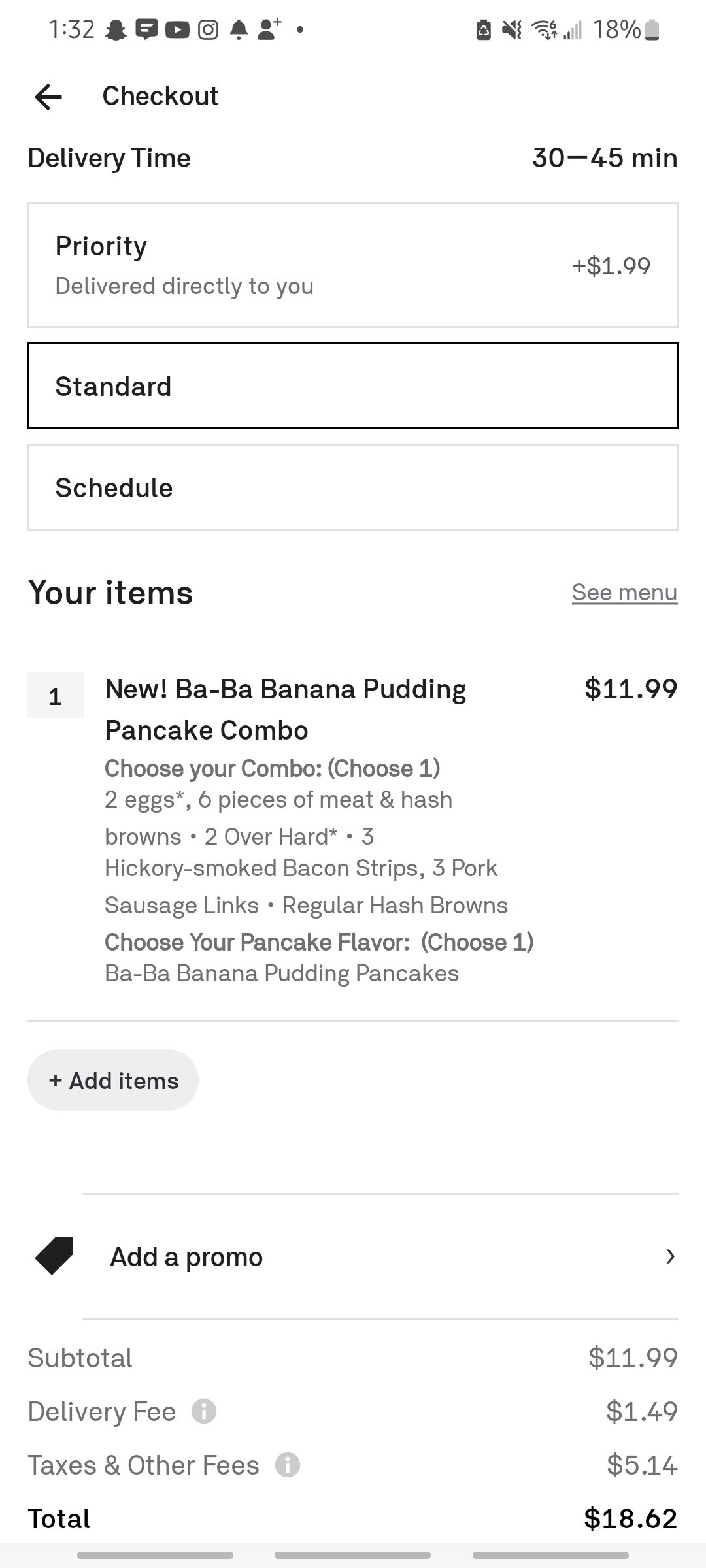The image displays a smartphone screen showing a detailed checkout process. In the top left corner, the clock indicates the time is 1:32. Surrounding the clock are various icons, including YouTube, notification bells, and more. On the right side, the status indicators display a Wi-Fi signal, a muted speaker, a low battery at 18%, and a network signal.

The main focus of the screen is a food delivery order in progress. The user has selected standard delivery, with an estimated arrival time of 30 to 45 minutes. The ordered item is a Baba Banana Pudding Pancake Combo, priced at $11.99. Additional charges include a delivery fee of $1.49, and taxes and other fees totaling $5.14, bringing the overall total to $18.62, prominently displayed in bold at the bottom.

The meal includes 2 eggs (over hard), 6 pieces of meat, hash browns, 3 hickory smoked bacon strips, and 3 pork sausage strips. The user has the option to choose their preferred pancake flavor to accompany the meal.